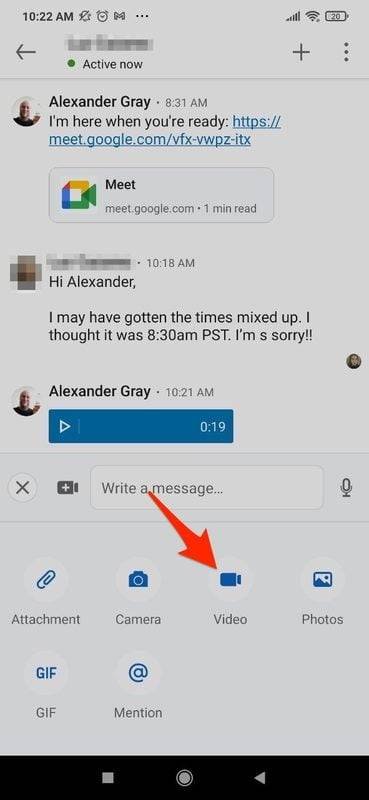In the screenshot captured at 10:22 a.m., we see a detailed communication exchange between two individuals. At the top, the bar displays indicators for Wi-Fi strength along with other notifications. A message bubble on the left, with a profile picture of Alexander Gray, reads, "I'm here when you're ready," followed by a Google Meet link: "meetgoogle.com." This message is marked as seen one minute ago with a Google Meet icon next to the link.

Adjacent to this, a blurred out response bubble reads, "Hi Alexander, I may have gotten the times mixed up, I thought it was 8:30 Pacific Standard Time, I'm sorry." Below this, another message from Alexander appears in a blue box, indicating a 19-second communication occurred. At the bottom, there is a large red arrow pointing towards the video icon next to the message input field. The attachment options available are labeled as attachment, camera, video, photos, GIF, and mention.